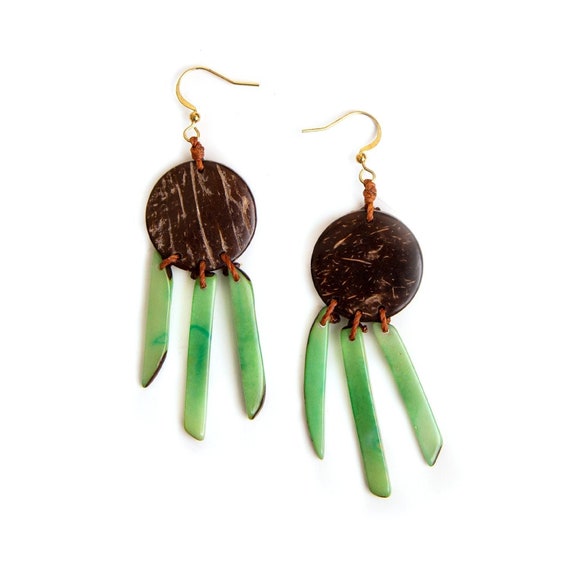Displayed against a clean, white background, this image features a pair of handmade, vintage-style earrings that could easily be found on a site like Etsy or eBay. The earrings are laid out on what appears to be a white table, with one earring positioned slightly higher than the other. 

Each earring is designed with a golden earring fastener that curves and hooks through the ear. The top part of the earrings features a large brown circular bead, adorned with light brown streaks that vary in direction, adding a rustic, handmade charm. Beneath the brown circle, three light green gemstones dangle like blades of grass, each of varying size and characterized by subtle dark green tints. These gemstones are attached to the brown bead with thin brown ropes or straw bands, accentuating the handcrafted aesthetic.